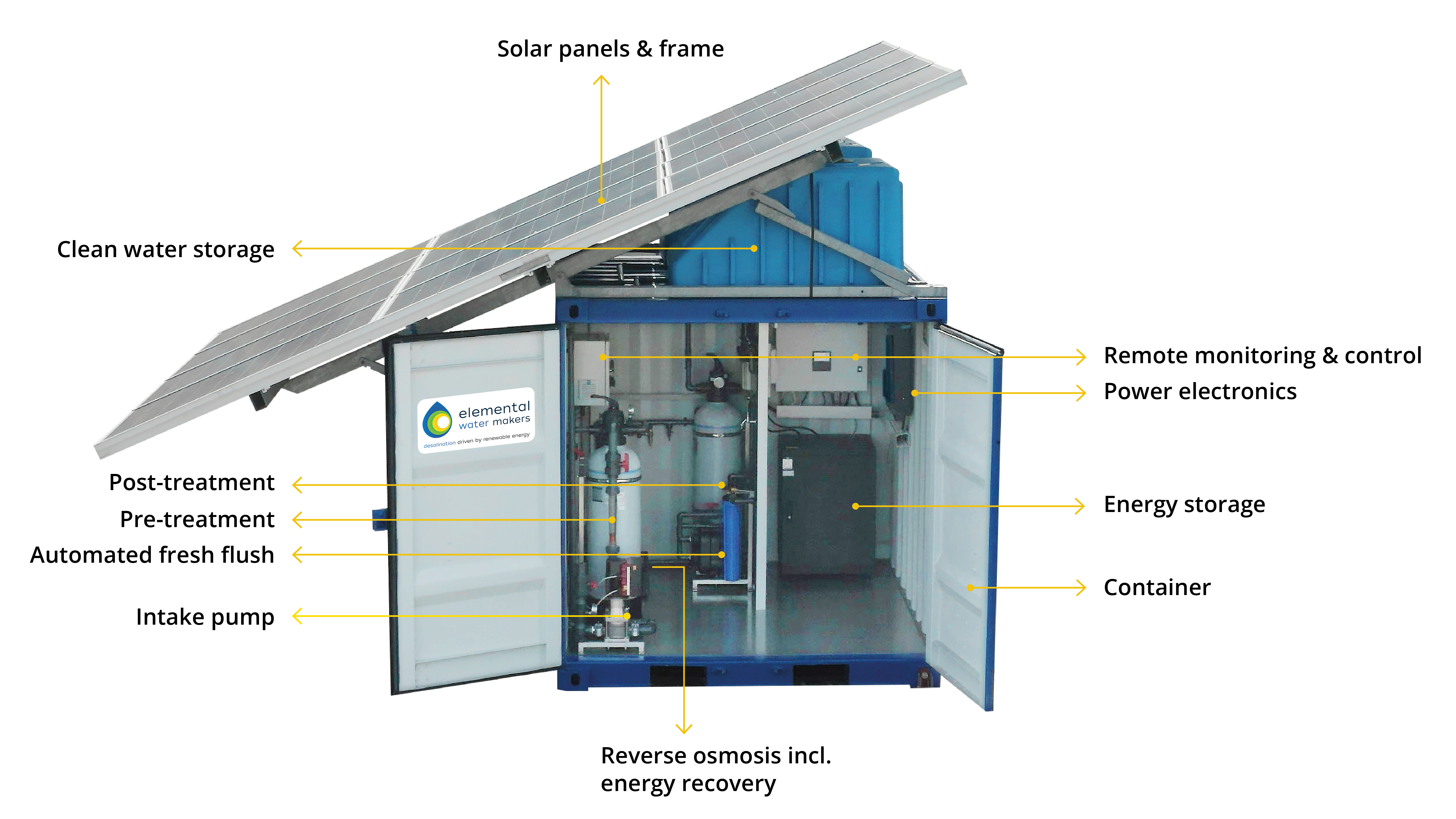This detailed diagram illustrates an Elemental water maker, designed for eco-friendly water and energy management. The top section of the image showcases solar panels mounted on a frame, which span from the upper right to the lower left. Directly beneath the solar panels is a clean water storage area, enclosed in a blue container. Below this, we see the open doors of a storage container, revealing the components vital for the system's operation. These include an intake pump, pre-treatment and post-treatment units, reverse osmosis system with energy recovery, energy storage, power electronics, automated fresh flush apparatus, and remote monitoring and control systems. The entire setup is meticulously labelled, highlighting its functionality and eco-friendly design for those looking to adopt green technologies.